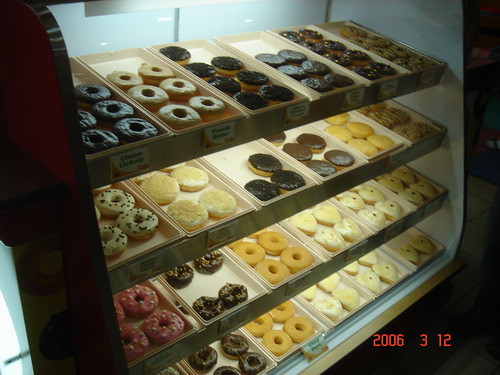The color photograph, dated with an old-school orange stamp reading "2006-3-12" in the bottom right corner, captures a close-up of a bakery display case brimming with an assorted selection of doughnuts. The image has a dark tone overall, but the doughnuts and their crates appear brighter due to the white illumination beneath each shelf. The display features multiple horizontal racks slightly angled forward for better visibility. Each rack holds a variety of doughnuts, with some sections completely filled while others have noticeable gaps where doughnuts have already been sold.

The doughnuts come in a myriad of flavors and types. Predominantly ring-shaped with holes, there are also fully rounded doughnuts without holes. The selection includes pink-iced doughnuts adorned with multi-colored sprinkles, white doughnuts sprinkled with chocolate chips, plain ring doughnuts, and various others with milk chocolate dipped tops. There's mention of more specific flavors such as maple dip, chocolate dip, Boston cream, and coconut dip. The doughnuts are organized into four distinct rows, each row further divided into six sections, featuring an array of cake doughnuts, glazed doughnuts, frosted doughnuts, and sprinkle-topped varieties.

As a tightly cropped image, it focuses solely on the doughnuts and their display, with no background or additional text visible except hints of signs indicating the doughnut flavors. The photo evokes a sense of nostalgia and hunger, reminiscent of popular doughnut shops like Dunkin’ Donuts or Tim Hortons.